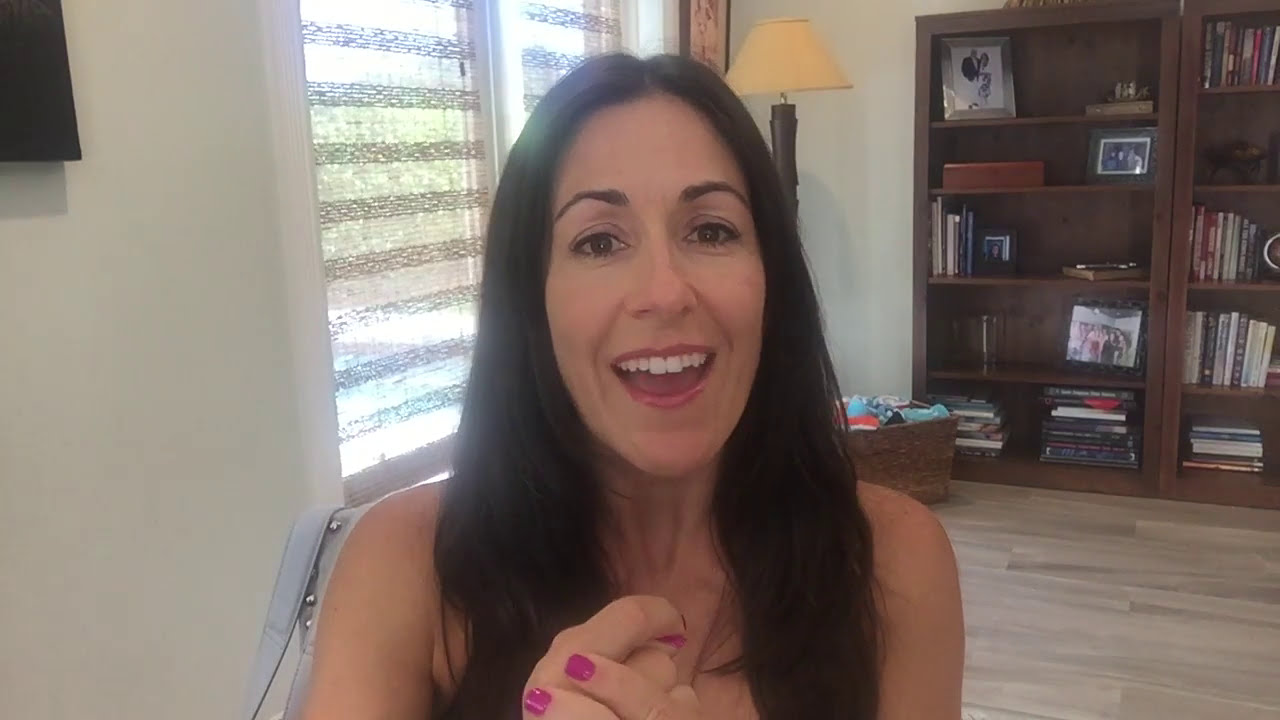In this detailed, color photograph, the central subject is a light-skinned woman in her late 20s or early 30s, captured mid-expression during what appears to be a Zoom or Skype call. She has a vibrant smile, with eyes that are lit up and animated, exuding excitement. Her long dark hair, parted down the middle, cascades past her shoulders. Her hands, adorned with short, lilac-pink nails, are clasped together below her neckline, near her chest.

The woman is seated, wearing a beige vest or halter top, though her attire is mostly obscured, suggesting a natural and possibly casual look for a video call. Her slightly parted lips show traces of slight red lipstick, reinforcing her lively demeanor as she engages passionately, possibly in mid-speech or in response to good news.

Behind her, the room is warmly lit by natural sunlight filtering through rattan blinds that cover a window, providing a shaded yet naturally bright ambiance. Bookcases flanking her sides are made of dark wood, each with four shelves sparsely filled with books, framed photographs, and other objects, adding a personal and lived-in touch to her space. In the corner of the room, a standing lamp with a yellow shade and brown post stands beside a wicker basket, which holds some towels or blankets. This background, featuring both a window with rain-spattered panes and cozy elements, forms a rich setting that complements her expressive and dynamic presence.